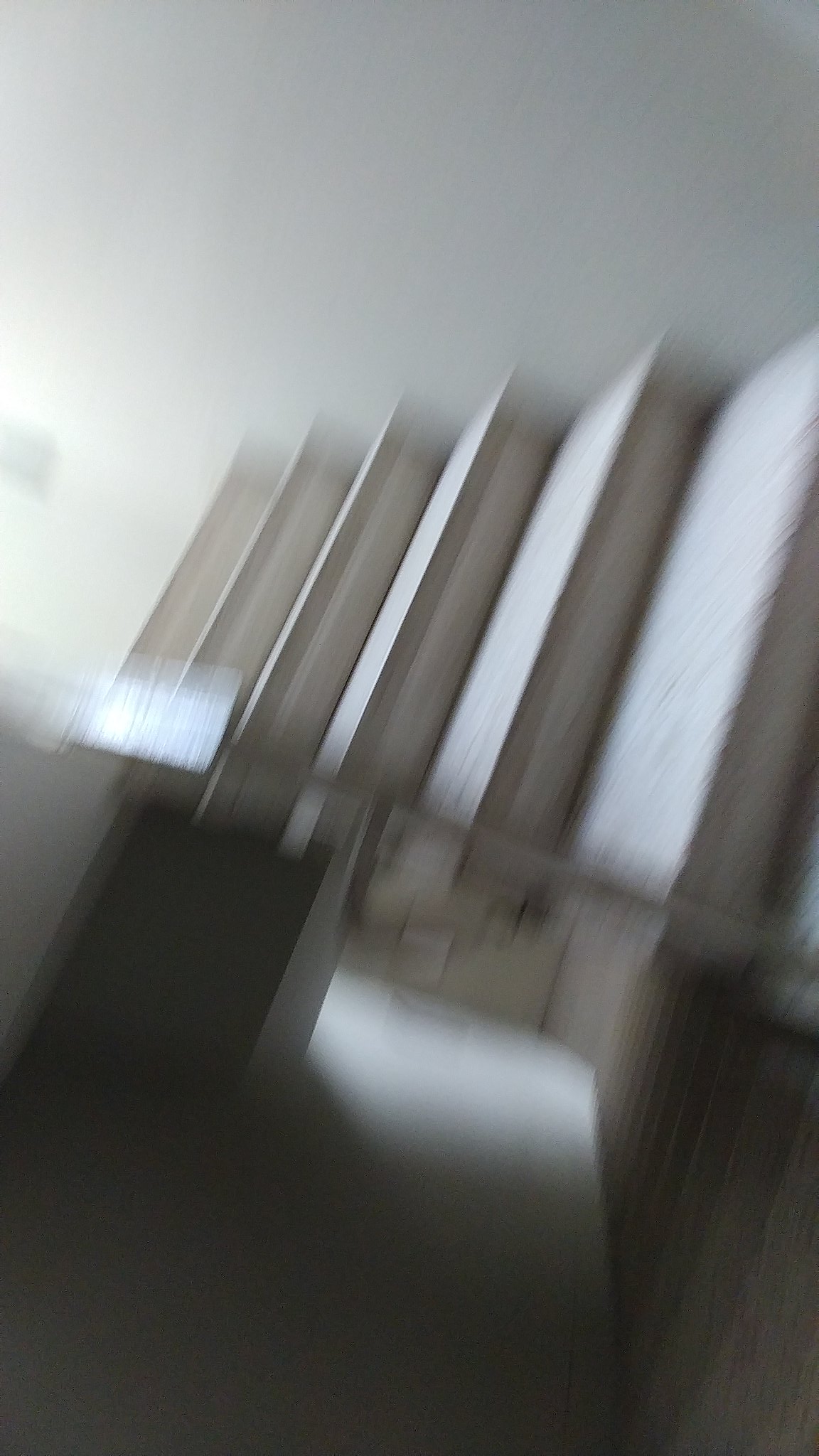This is a photograph, though heavily blurred, depicting a stairway inside a predominantly white home or building. The camera angle appears skewed, as if taken from the middle section of the stairs, causing the staircase to look slightly tilted. In the lower part of the image, some stairs descend into darkness, while in the upper part, stairs ascend brightly illuminated by what seems to be natural light. The walls surrounding the staircase are white, and the stairs themselves are either light beige or white. The stairway includes a landing, with flights of stairs positioned side by side, giving an impression of an upward and a downward trajectory. Whites and grays dominate the overall color scheme, contributing to a stark, monochromatic aesthetic. No other details or objects are discernible in the image due to the blurriness.